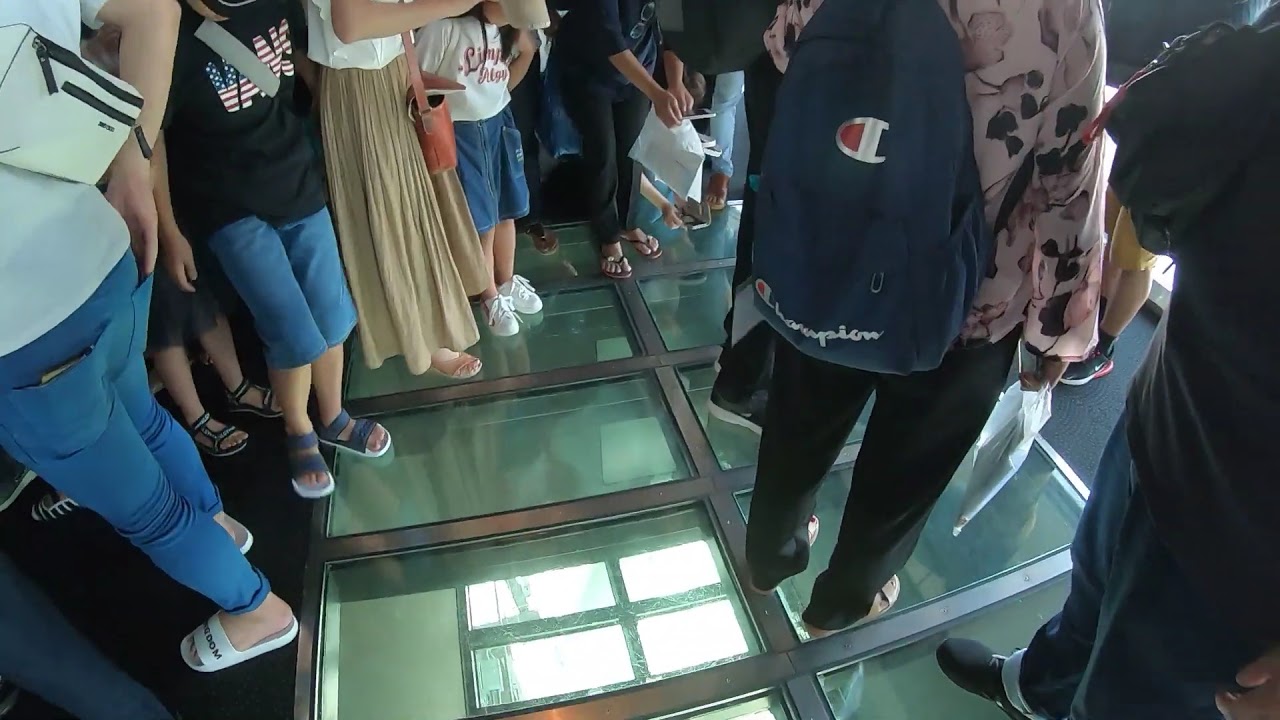This detailed image captures the interior of what appears to be a glass-floored observation area, potentially in a skyscraper, offering a clear view down to the lower level. The glass floor is made up of large, rectangular panels and is set within a frame. The reflective and transparent nature of the glass allows for the visibility of structures below, as well as reflections, suggesting a sunny day outside. 

The main focus of the photo is the lower halves of 11 to 13 people standing on the glass floor, with no faces visible. Their attire is varied - some wear pants, shorts, or skirts, and most are in sandals or slippers, although one girl is noted to be wearing white shoes. Notably, to the right of the image, a woman is carrying a navy blue Champion backpack, identifiable by the red, navy, and white logo and the word "Champion" written in cursive at the bottom. To the left, a person is noted to have their hand in their pocket, wearing blue jeans, a white shirt, and another individual is identified wearing a black t-shirt with a Vans logo designed like the American flag, along with blue trousers and sandals.

Overall, the photo captures a unique perspective through the glass floor, highlighting the diverse attire and accessories of the people present.